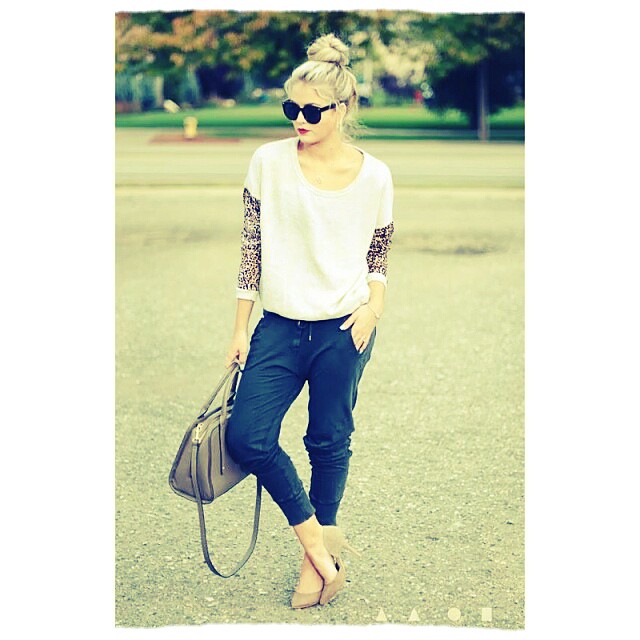In this stylish throwback image reminiscent of the 80s, a young, attractive blonde woman models in a setting that looks like a public park with blurred grass and trees in the background. Her blonde hair is elegantly swept up into a large bun, and she sports large, Ray-Ban-like sunglasses that add a touch of mystery to her look. Red lipstick accentuates her face, enhancing her striking appearance.

She wears a cream-colored, loose-fitting three-quarter sleeve top with a distinctive black-and-white patterned design on the sleeves. Her outfit is completed with blue capri sweatpants that have a comfortable yet chic vibe. A fashionable bracelet decorates her right wrist, matching her tan suede high spike heels. She carries a large, fashionable handbag in her right hand, while her left hand rests partially inside her pocket.

In a casual yet poised stance, she has one leg slightly bent, crossing the foot over the other at the ankle, which pushes her knee slightly outward against the handbag. This image, focused on her, captures an aura of modern elegance with a nostalgic twist, making her appear to be a model in a fashion advertisement, evocative of the 80s or very early 90s.